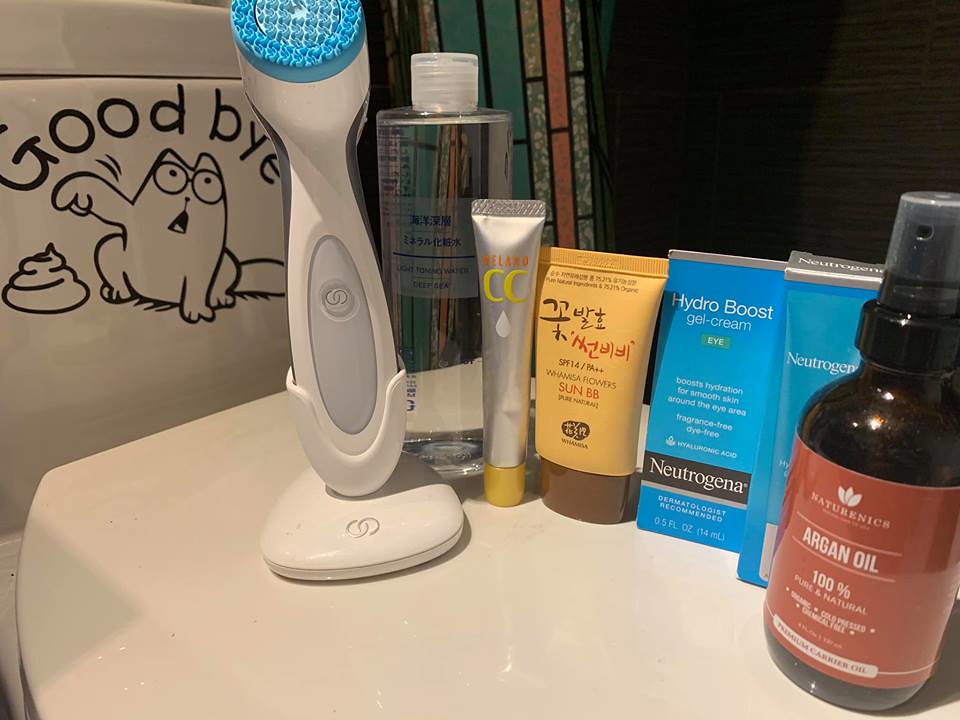This image showcases an assortment of bathroom essentials meticulously arranged on a plastic table. 

On the right, a dark bottle with a maroon label contains argan oil spray, standing prominently in the foreground. Just behind it, there are two distinct Neutrogena products, easily identified by their turquoise blue boxes adorned with white lettering. The first Neutrogena item is clearly labeled as Hydro Boost Gel Cream for Eyes.

Adjacent to these, a BB cream with a brown cap and a slightly yellowed squeeze bottle body is noticeable. Beside it is a slender silver tube marked Bolaro CC, complemented by a yellow lid, indicating it is a CC cream.

Near these items, there's a container filled with a clear liquid, equipped with a squirt nozzle; the label bears Asian characters, though its exact purpose remains unclear. Lastly, an electronic facial scrubber with blue bristles completes the assortment, likely powered by batteries, hinting at a more technologically advanced skincare tool.